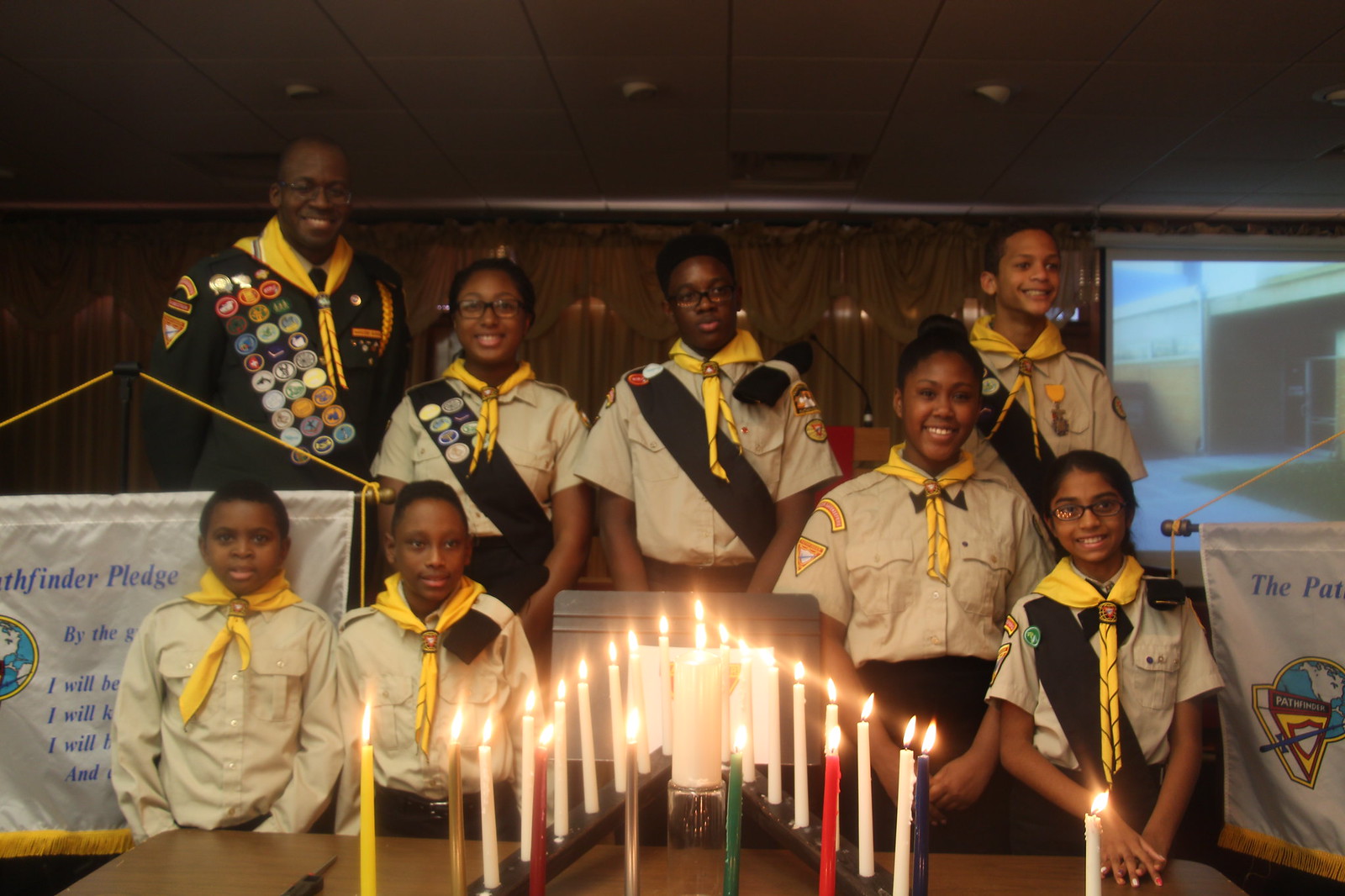In the photograph taken inside a small building with a tiled roof, a diverse group of eight individuals stands behind a wooden table, prominently featuring a tall, slanted menorah-like candle arrangement. The triangular display is filled with lit candles, predominantly white, with a multicolored front row: yellow, white, red, silver, green, red, white, blue. The candle holder appears to form a staircase effect, with candles ascending and descending symmetrically.

The group consists of seven children and one adult, all dressed in tan Scout-like uniforms. The children wear yellow scarves around their necks, with some sporting sashes adorned with various patches. Particularly notable is the girl on the top left with the most patches (eight), indicating her seniority or achievements. Just beside her, the man, likely the Scout leader, is attired in a darker brown uniform with a yellow scarf and a heavily decorated sash boasting upwards of 20 badges.

The scene, likely a gathering of a Scouting or similar youth organization, has an air of ceremony and camaraderie. To the right-hand side of the room, there is an overhead projector screen and partially visible flags, suggesting a formal setting. The children and their leader are all smiling, looking towards the right of the frame, creating a warm and engaging atmosphere.